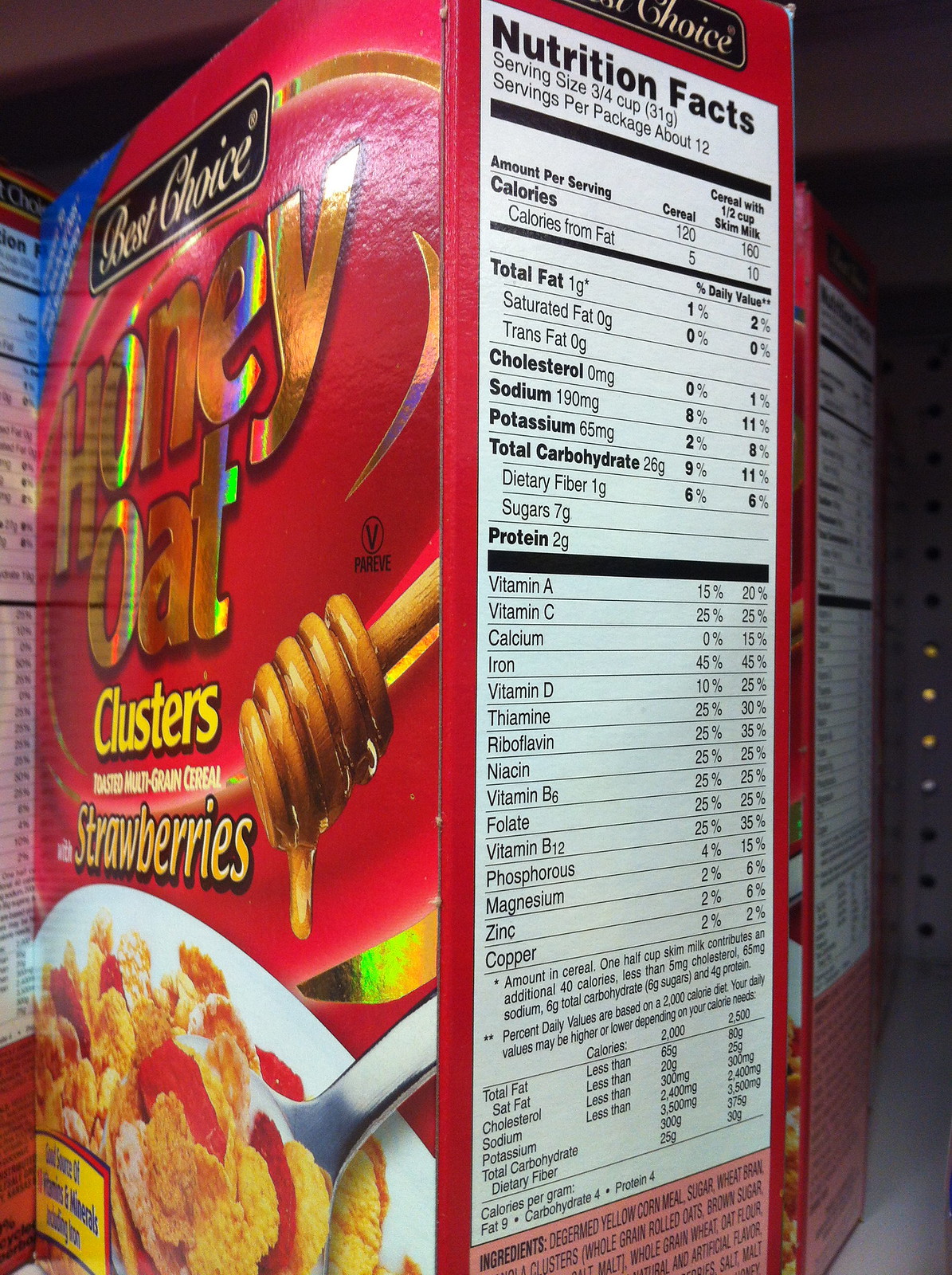This is a photograph taken in portrait mode of a box of cereal, primarily showcasing the right side panel and partially the front. The box is mostly bright red with reflective gold and brown lettering that reads: "Best Choice Honey Oat Clusters." Smaller text indicates the cereal contains "Strawberries." The front of the box features an image of a bowl of cereal with oat flakes, strawberry pieces, and a honey stick drizzling honey. The right side panel, prominently displayed, is a white rectangular box with black text detailing the Nutrition Facts, including serving size (¾ cup or 31 grams), calories, fat, cholesterol, sodium, potassium, total carbohydrates, proteins, and various vitamins and minerals. At the bottom of the nutrition label, part of the ingredient list is visible but partially cut off.